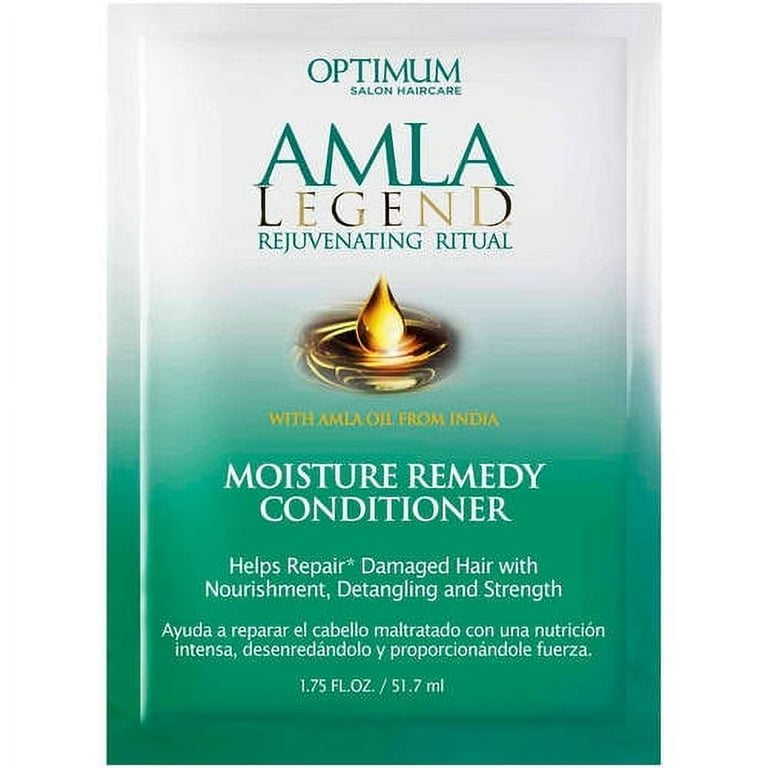The image features a rectangular, single-use packet of Optimum Salon Haircare's 'AMLA Legend Rejuvenating Ritual.' The packet is predominantly white at the top, with a gradient that transitions into a light aqua green at the bottom. The front of the package prominently displays 'Optimum Salon Haircare' at the top, followed by 'AMLA Legend Rejuvenating Ritual' written in black and gold. Below this, an image of a golden liquid drop falling into a pool of gold is visible. Accompanying text in green and yellow states 'With AMLA Oil from India.' Further down, in white text, it reads 'Moisture Remedy Conditioner', highlighting benefits such as helping to repair damaged hair with nourishment, detangling, and strength. Additionally, there is text in a foreign language, presumably 'Adura Repaira.' The packet's volume is noted at the bottom as '1.75 fluid ounces / 51.7 milliliters.' The packaging is designed for easy tear opening, with seams along the edges.